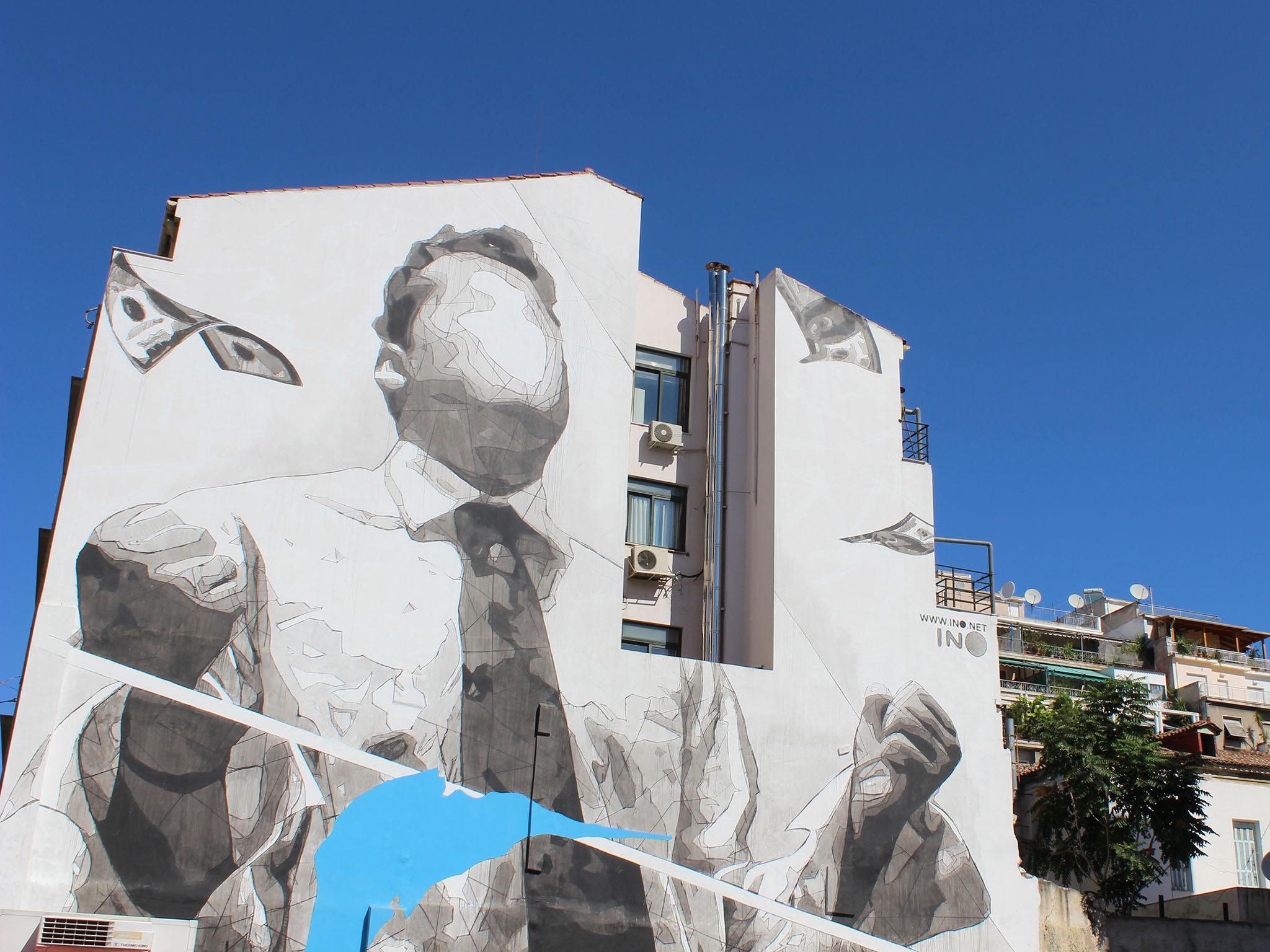The image depicts a tall building with a unique, irregular facade featuring a recessed middle section and varying heights between its left and right sides. It is primarily concrete with three stories of windows and AC units attached. A large, black-and-white mural adorns its side, showcasing a faceless man with short brown hair, a white-collared shirt, and a dark tie with faded colors. His fists are raised to his sides as if in a stance of determination or defiance. Several dollar bills appear to be falling around him, some positioned near the upper left and others cut off by the building's edge. The mural is visually intersected by a white line that oddly dissects his right hand and extends downwards and rightwards through the composition. Additionally, there is blue paint marking the figure, particularly around his tie. Surrounding this mural-clad building is a complex with satellite dishes and patio-covered condominiums or apartments. The background features a blue sky, a tree, and more buildings, contributing to the vibrant, urban atmosphere of the scene.